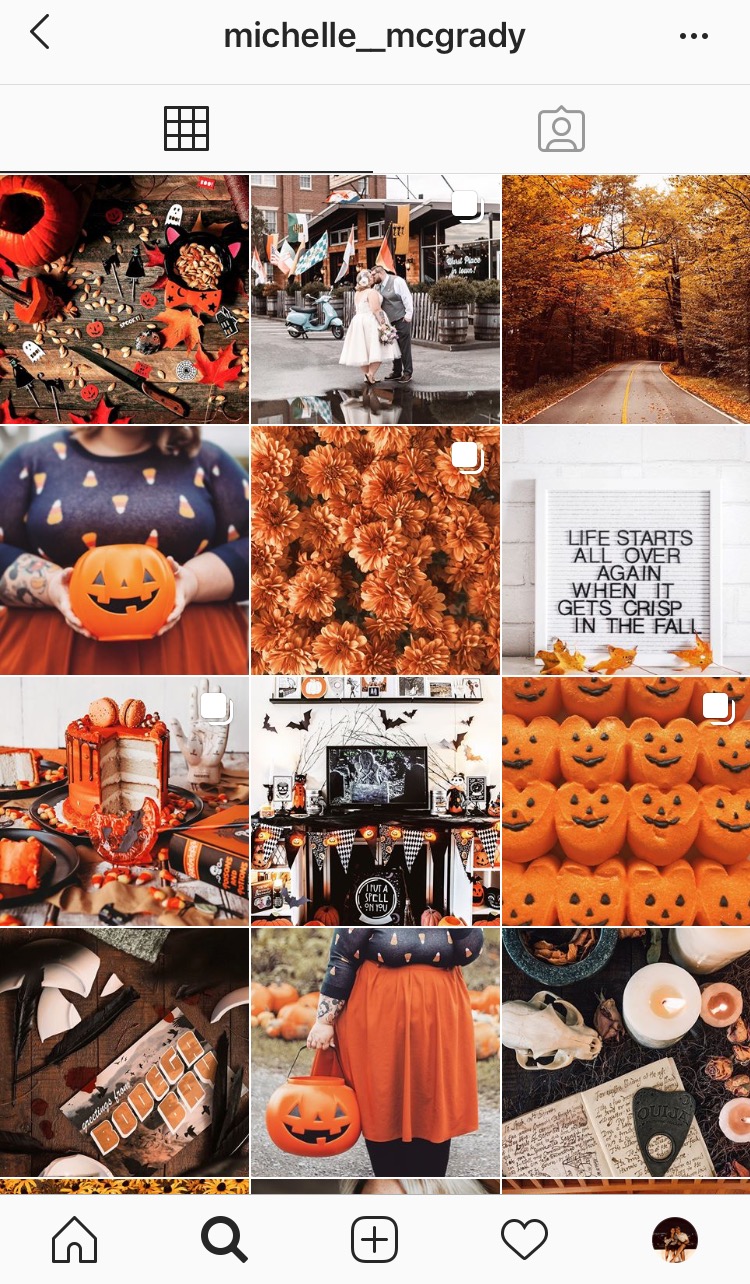The image appears to be a screenshot from a smartphone, displaying a gallery of square photos arranged in four rows with three pictures per row. At the very top of the screen, there is a gray background featuring an arrow pointing to the left on the far left side, followed by the username "Michelle_McGrady." On the far right, there are three vertical dots, indicating additional options or settings.

Underneath this header, there are two icons: one on the left showing a grid of three rows of three squares, and another on the right depicting a generic person silhouette graphic. Each of the twelve images in the gallery has a Halloween or pumpkin theme, characterized by predominantly orange and brown hues.

In the top right image, there is a scenic roadway lined with trees sporting vibrant orange and yellow leaves. Moving to the second row, the far-left image showcases a woman in a blue shirt adorned with candy corns, holding a pumpkin with a black carved face. Immediately to the right of this, there is a picture of orangish-brown mums in full bloom.

On the fourth row, the middle image again features the woman in the blue candy corn shirt. This time, she is wearing an orange skirt and holding the same pumpkin bucket at her side, completing the festive Halloween ensemble. The collection of photos exudes a warm, autumnal atmosphere, encapsulating the essence of the Halloween season.